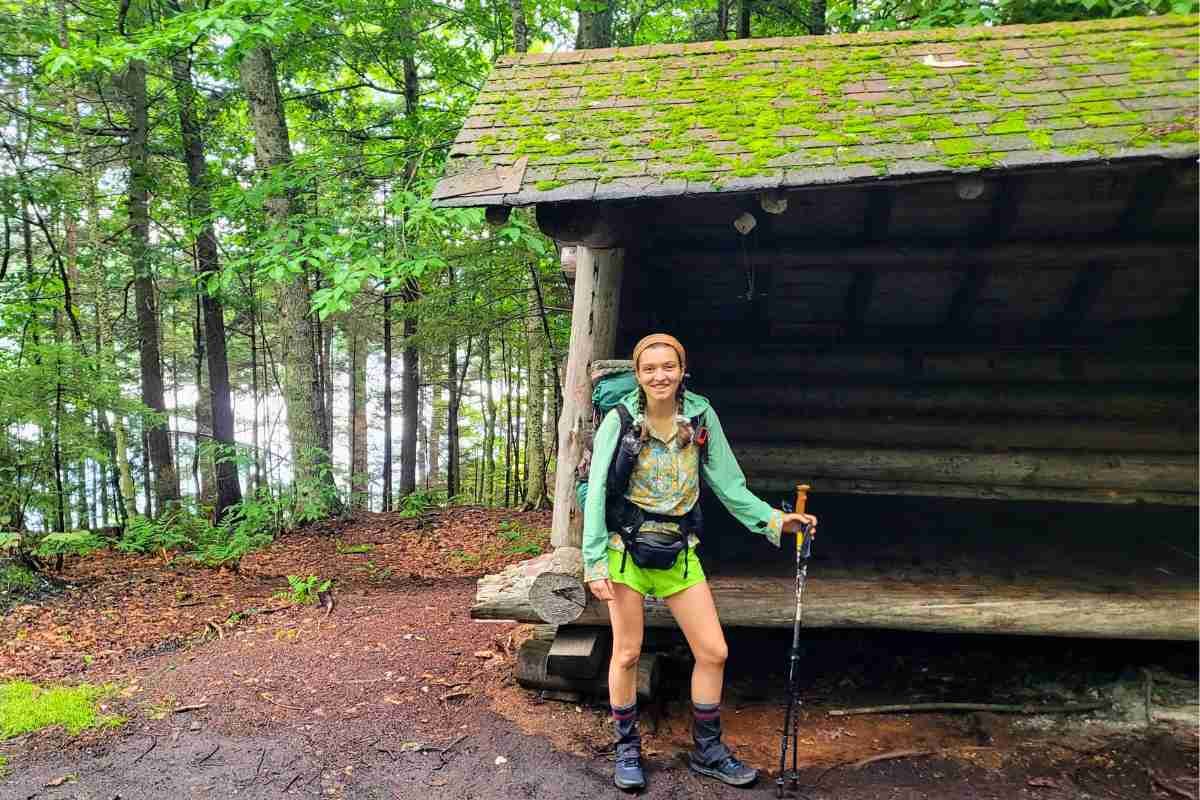The color photograph showcases a vibrant outdoor scene on a cloudy, possibly post-rainy day. The focal point of the image is a woman dressed in hiking gear, standing confidently in front of a rustic wooden structure. This log-built shelter, resembling a covered bench, features a roof adorned with bright green moss and appears slightly tilted to the right. The interior is dim, yet a bench made of logs can be faintly discerned through its open front.

The hiker is dressed in practical outdoor attire: dark hiking boots and socks, neon lime green shorts, and a pastel green jacket with a floral body. She carries hiker poles in her left hand and has a black fanny pack secured around her waist. A teal backpack is strapped to her back, equipped with essential hiking gear. Her medium-length brown hair is styled in two braids, and she wears an orange headband. The woman is smiling warmly at the camera.

Surrounding the wooden structure is a lush forest landscape. Tall, big green pine trees stretch toward the sky, with their leaves casting gentle shadows. The ground is wet and scattered with brown leaves, pine needles, small bushes, patches of grass, and stones. The background offers a distant view of a white, cloudy sky and what appears to be a hilltop or mountain. Trails wind through the forested area, leading toward a lake partially visible beyond the trees.

The overall scene captures a serene moment of nature and adventure, with the hiker ready to embrace the outdoors.